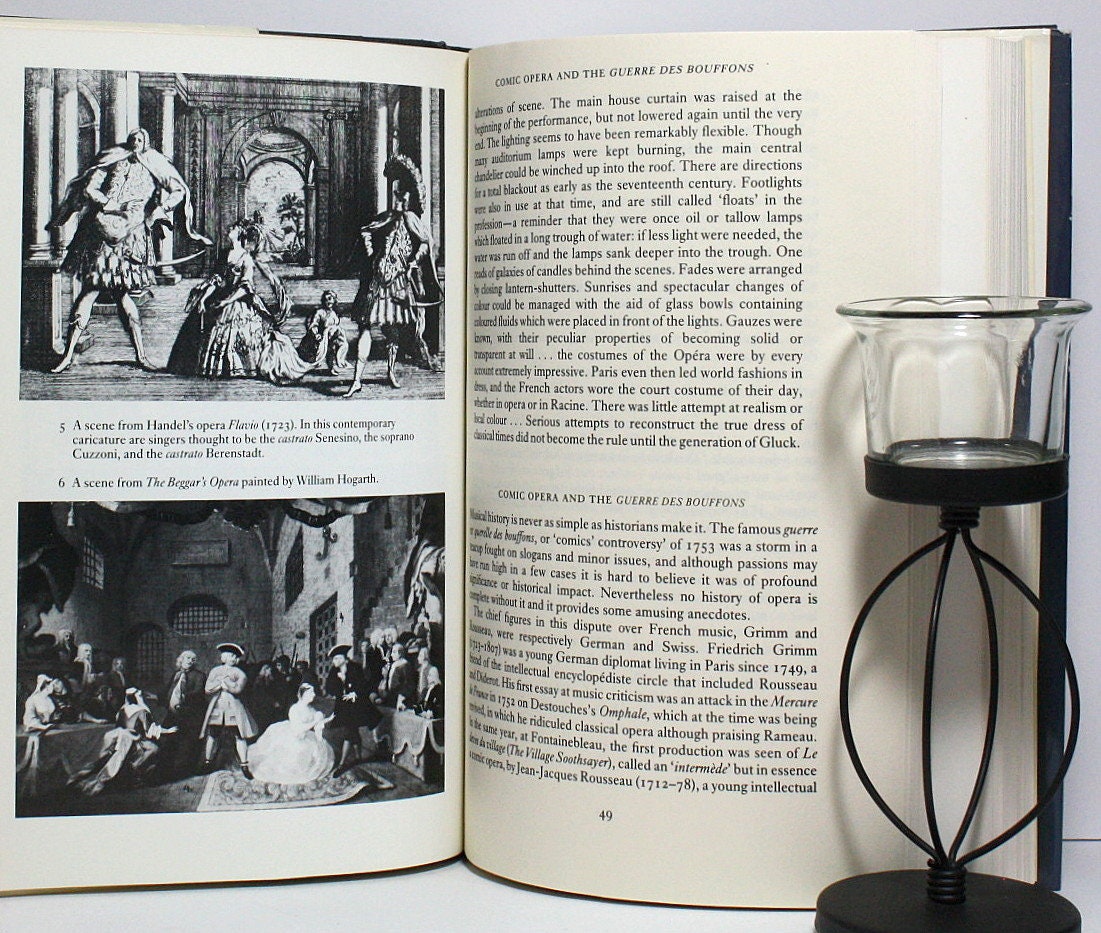The image shows an open book, titled "Comic Opera and the Guerre des Bouffons," propped up against an unseen surface. The book is open to pages 48 and 49. Page 48 features two hand-drawn, renaissance-era illustrations, labeled five and six, depicting scenes from Handel's opera, Flavio. The right-hand page, 49, contains detailed text, structured in two paragraphs at the top and likely two more at the bottom, explaining the history of certain plays and operas. To the right of the book, a black candle holder with a glass cup at the top helps in keeping the book open. The photograph appears to have been taken indoors.